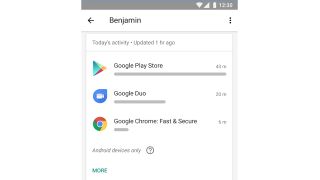The image depicts the screen of a device, characterized by low quality and low resolution, resulting in a blurry and pixelated appearance. In the upper right corner of the screen, there are icons for WiFi, cellular signal, and battery status next to the time displayed as 12:30. 

In the top left corner, a black left-pointing arrow is visible, while the name "Benjamin" is centered and clearly spelled out. On the far right of this section, a "more" icon consisting of three vertical black dots is present. 

Below these elements, a line of text, despite its blurry nature, reads: "Today's activity, update one hour ago." Further down, on the left side, the Google Play icon is noticeable, followed by the text "Google Play Store." Subsequently, "Google Duo" is displayed beneath the previous text.